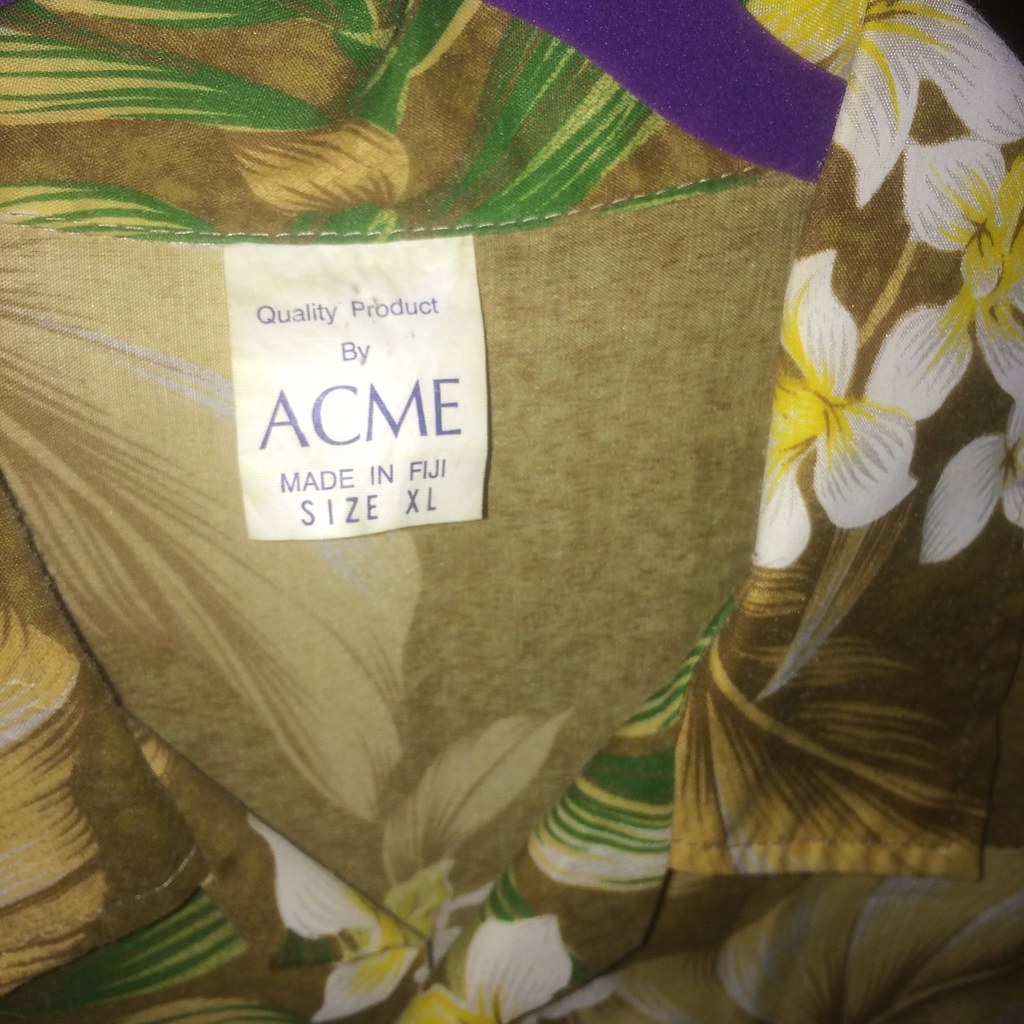This detailed photograph captures the interior label of a tropical Hawaiian-style shirt, vividly highlighting its intricate details. The fabric of the shirt, which radiates a rich golden hue, is adorned with an array of white and yellow flowers interspersed with verdant green leaves, exuding a vibrant and exotic aesthetic. Centrally focused in the image is the label, meticulously sewn into the collar of the shirt. The label, with its white background, prominently displays text in a distinctive purplish-black font that reads "Quality product by Akume, made in Fiji, size XL." The overall composition not only emphasizes the craftsmanship and details of the shirt but also subtly suggests its premium quality and tropical origins.